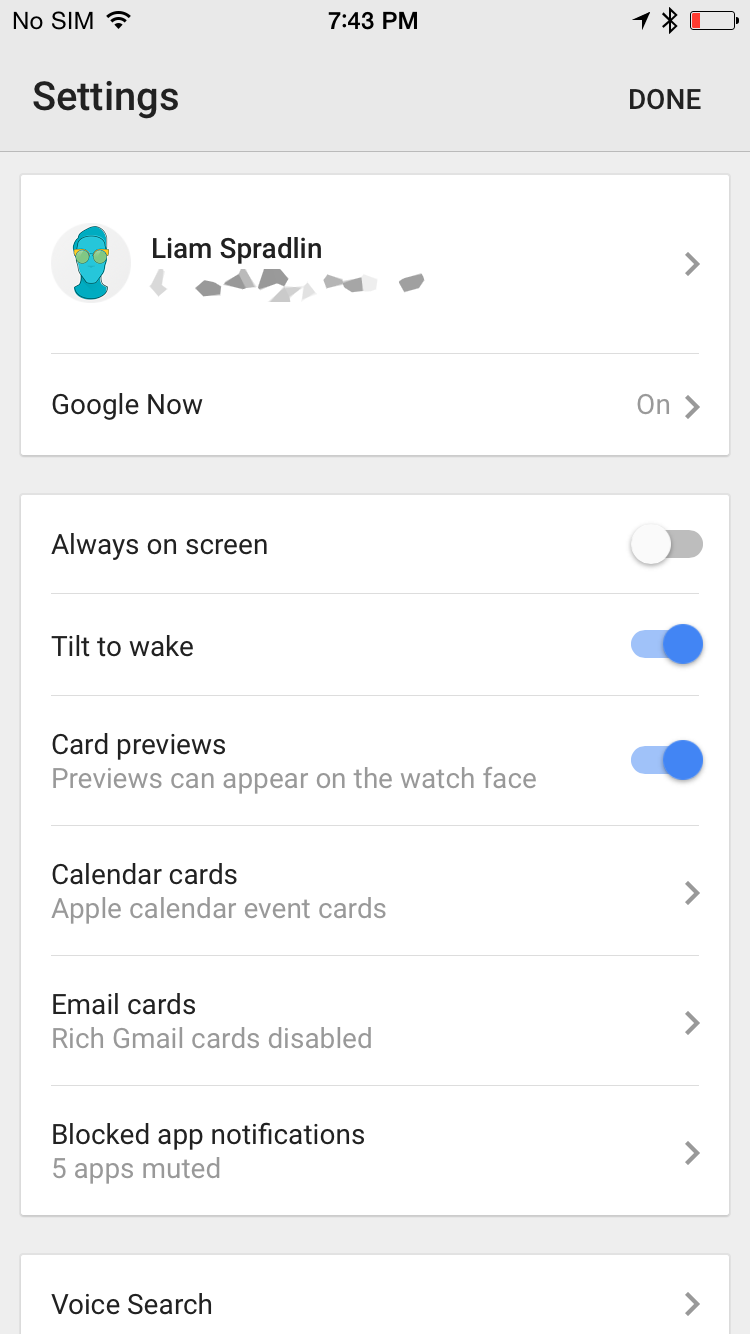In this image, we are looking at a settings page, likely from a smartwatch. At the top of the screen, indicators show that there is no SIM card installed, the time is 7:43, and the battery level is critically low, displayed in red. The main title of the settings page is prominently labeled with "Settings," and there is a "Done" button for exiting the menu.

Below the title, there is the user’s identification: "Liam Spradlin," accompanied by an animated avatar. The settings menu includes multiple options:
1. "Google Now" which is currently enabled.
2. "Always On Screen" which is disabled.
3. "Tilt to Wake" which is enabled.
4. "Card Previews," which allows previews to appear on the watch face, and is enabled.
5. "Calendar Cards" specifically for Apple Calendar event cards, which can be accessed by tapping the option.
6. "Email Cards," where rich Gmail cards are disabled.

Further down, there is an option for "Blocked App Notifications," indicating that five apps have been muted. At the bottom of the settings page, there is an option for "Voice Search," which can be activated.

Overall, the image provides a detailed view of the various customizable settings available on the smartwatch, catering to user preferences for notifications, screen behavior, and information display.